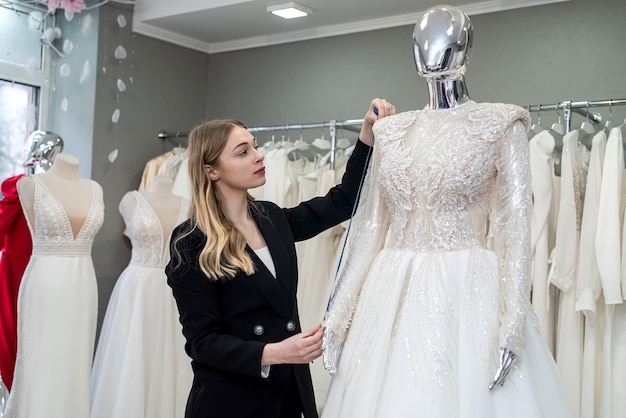This detailed image presents the interior of a sophisticated bridal studio, featuring a central focus on a stunning cream-colored wedding dress displayed on a shiny silver mannequin. The dress is elaborately adorned with ornate beadwork and lace details, accompanied by long sleeves. A meticulous woman with medium-length blonde hair, light skin, and dressed in a black double-breasted blazer over a white shirt, is carefully measuring the length of the gown's arm. The backdrop highlights a rack of various other wedding dresses and two additional, less ornate white mannequins donning simpler bridal gowns. To the far left edge of the frame, a glimpse of another silver mannequin wearing a red dress is barely visible. The studio’s ambiance is accentuated by its plain gray walls, a square white ceiling light, and a small bit of window with a hint of a white mobile hanging from the ceiling. The impeccably organized space, with its ceiling lighting, highlights the meticulous designs of the wedding dresses, enhancing the shop's elegant atmosphere.